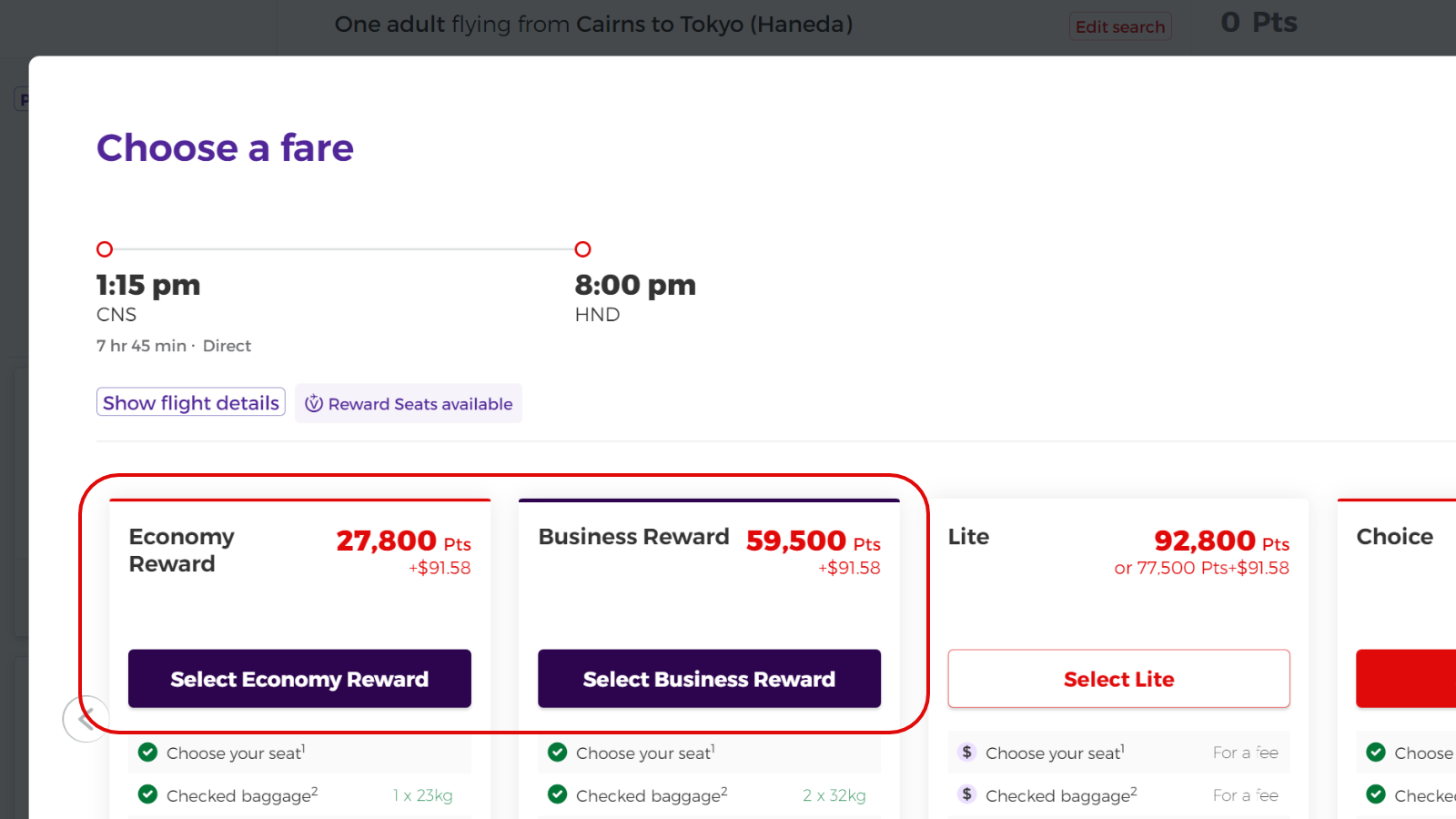The image appears to be a cropped screenshot from a desktop PC or laptop. It focuses on a pop-up overlaying a darkened background, suggesting it was triggered by an action on a website. The visible portion of the pop-up has a white background with the header "Choose a fare" in purple text located at the top left corner. 

Centered on the pop-up, there is a graphical representation of a flight itinerary featuring two circles connected by a gray line. The first circle on the left reads "1:15 PM, CNS, 7 hour 45 minute direct," indicating the departure time and location. The line extends to a second circle on the right that reads "8:00 PM, HND," indicating the arrival time and location.

Below this graphical itinerary, there are two pricing options outlined in a red box. The first option is labeled "Economy Reward," priced at 27,800 points plus $91.58. The second option is labeled "Business Reward," priced at 59,500 points plus $91.58. The screenshot is cropped, cutting off the bottom and right edges, preventing a full view of the pop-up.